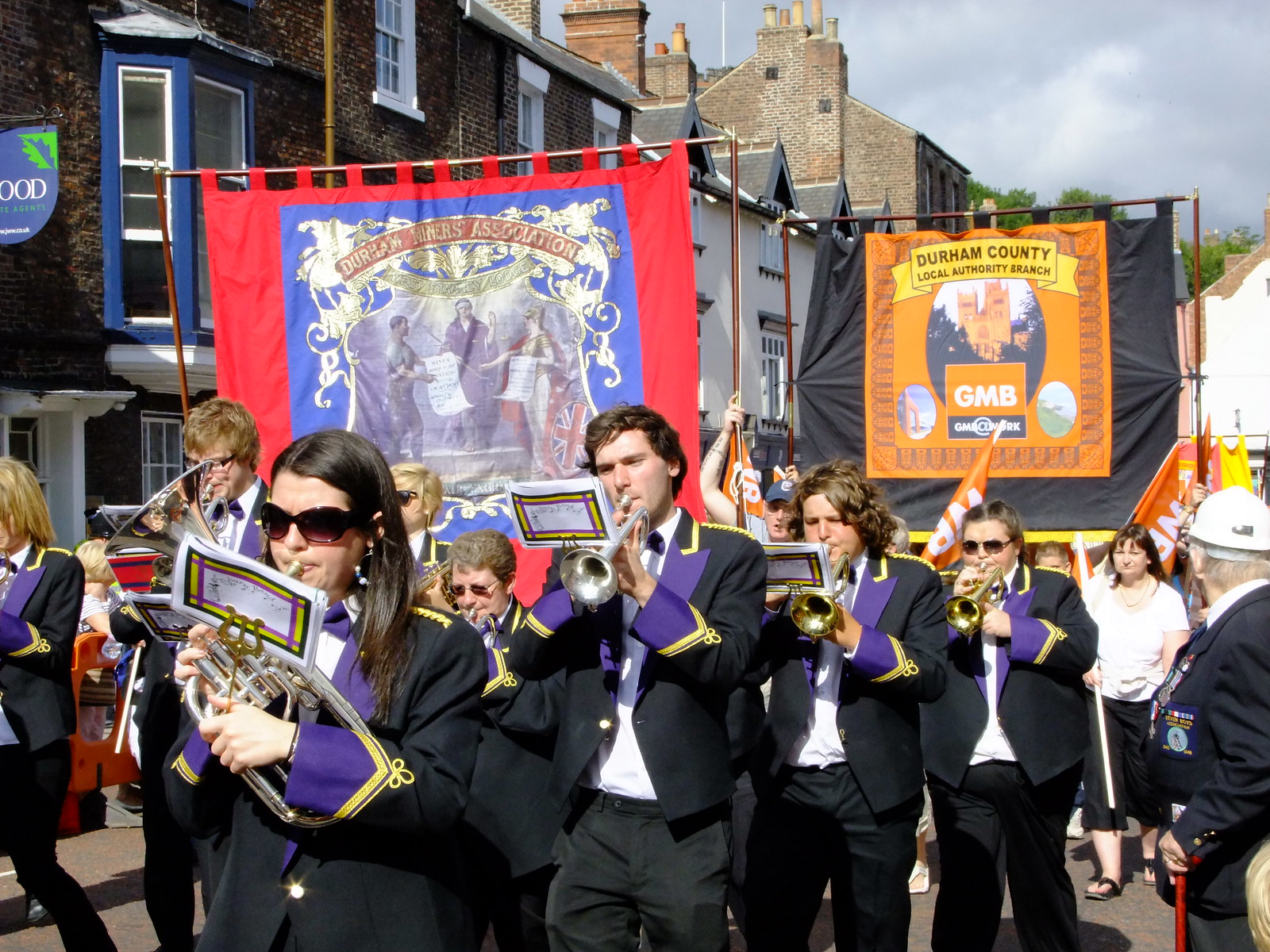The image depicts a formal parade featuring a marching band in a quaint English town. The band members, around a dozen in number, are dressed in elegant black uniforms resembling nautical attire, with purple bow ties, elaborate purple and gold cuffs, gold shoulder decorations, and collars. They are playing an array of brass instruments, including trumpets, French horns, and a tuba, with their music sheets clipped to the instruments. The parade proceeds down a street lined with old buildings, some made of brick and others with white siding, evoking a historical ambiance.

In the background, participants carry prominent banners. The closest banner, with a red background, features a detailed painted crest showing a man pointing to a scroll, a soldier holding a scroll, and a lady justice with a shield bearing the British flag. This banner is associated with the Durham Miners Association, as indicated by a scroll at the top. Another banner in the procession is orange and bears an illustration of a castle, labeled "Durham County Local Authority Branch" in a yellow banner. The banners enhance the traditional and local significance of the parade, likely taking place in a historic locale within the British Isles. The combined elements of the uniforms, brass band, and distinctive banners create a vivid scene of cultural and community celebration.